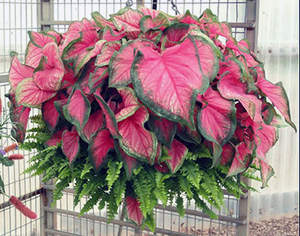The image shows a small square photograph featuring a beautiful hanging plant system against a backdrop of white, clear plastic corrugated greenhouse siding. The plant is suspended from a metal rack via small chains that extend out of the image. The top section of the plant showcases a Callidome bicolor with striking, large, heart-shaped leaves that are predominantly pink with dark green borders. These vibrant leaves are especially abundant on the left and right sides, with an especially large one in the middle slightly to the right. The lower portion of the plant features regular fern leaves that are lime green and appear to jut out with small spikes along their borders. On the ground, you can see brown, dirty river rocks localized to the bottom right corner. The background also reveals a metal cage just to the right of the plant, with some plant leaves extending past its edge. The serene and orderly setting within the greenhouse emphasizes the elegance of the hanging plant system and the contrasting textures of the Callidome bicolor and the fern.